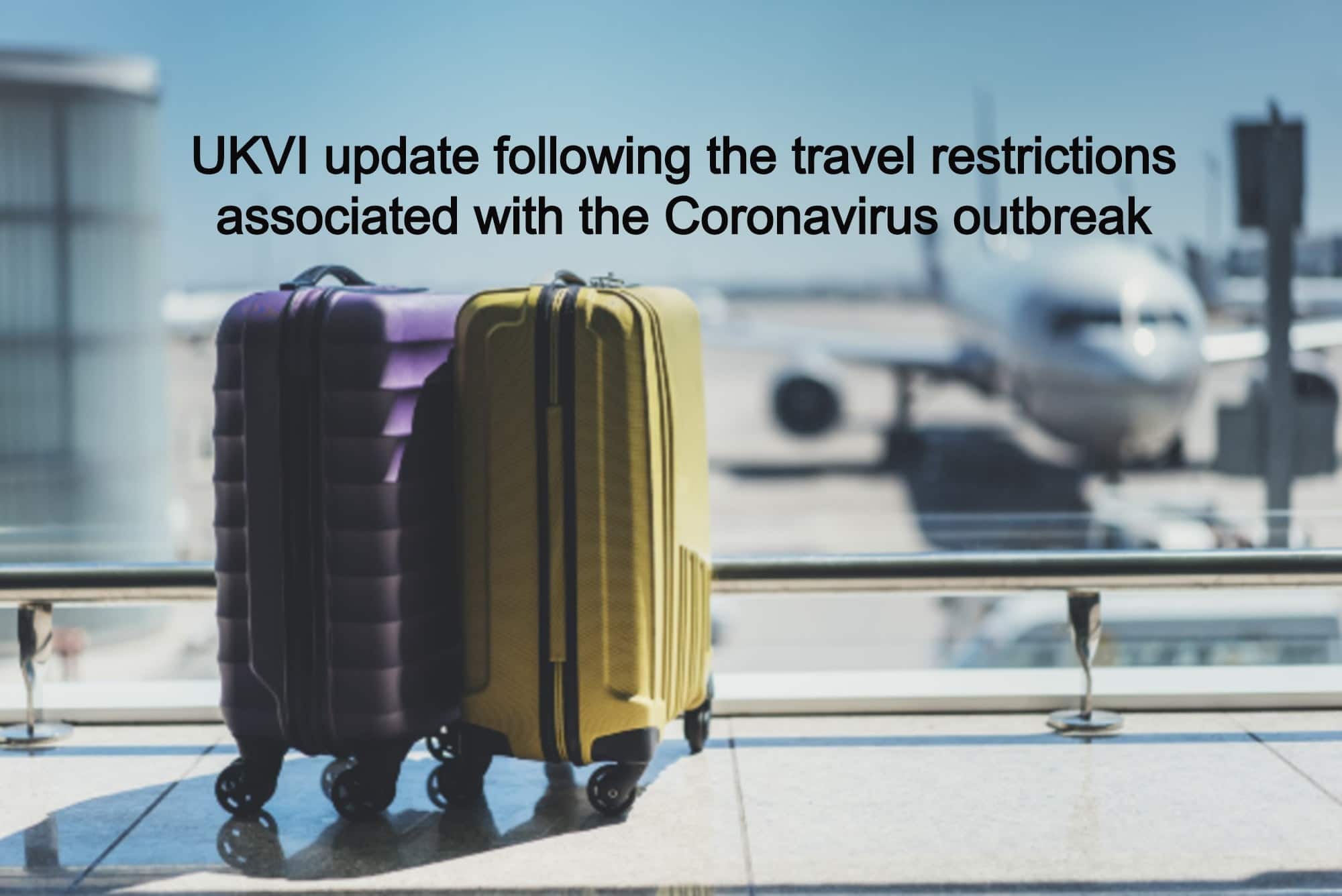In the foreground of this wide rectangular image, two focused suitcases dominate the scene. The suitcase on the left, adorned in a rich purple hue, is partially obscured by the one on the right, which gleams in gold. Both suitcases, equipped with black wheels and textured designs, sit on the floor inside what appears to be an airport terminal. The purple suitcase features horizontal textured lines, while the gold one sports vertical textures near its base. Black handles top each suitcase, and sunlight filters through a nearby window, casting shadows that extend towards the bottom left corner of the image.

In the midground, a low horizontal chrome bar spans the width of the frame, separating the foreground from the distant view beyond the window. The background is a blur of blue skies and architectural elements. On the right side, a silver plane faces forward, bathed in sunlight that creates reflective highlights on its surface. The left side of the background features a building, both elements contributing to a palette of blue and gray tones.

Above the suitcases and extending towards the airplane, black text overlays the image. The top line reads "UKVI" in bold capital letters, followed by a secondary line in lowercase: "update following the travel restrictions." Beneath this, the text continues: "associated with the Coronavirus outbreak," with the 'C' in Coronavirus capitalized. The text placement draws attention to the urgent travel advisory while blending seamlessly into the composition of the image.